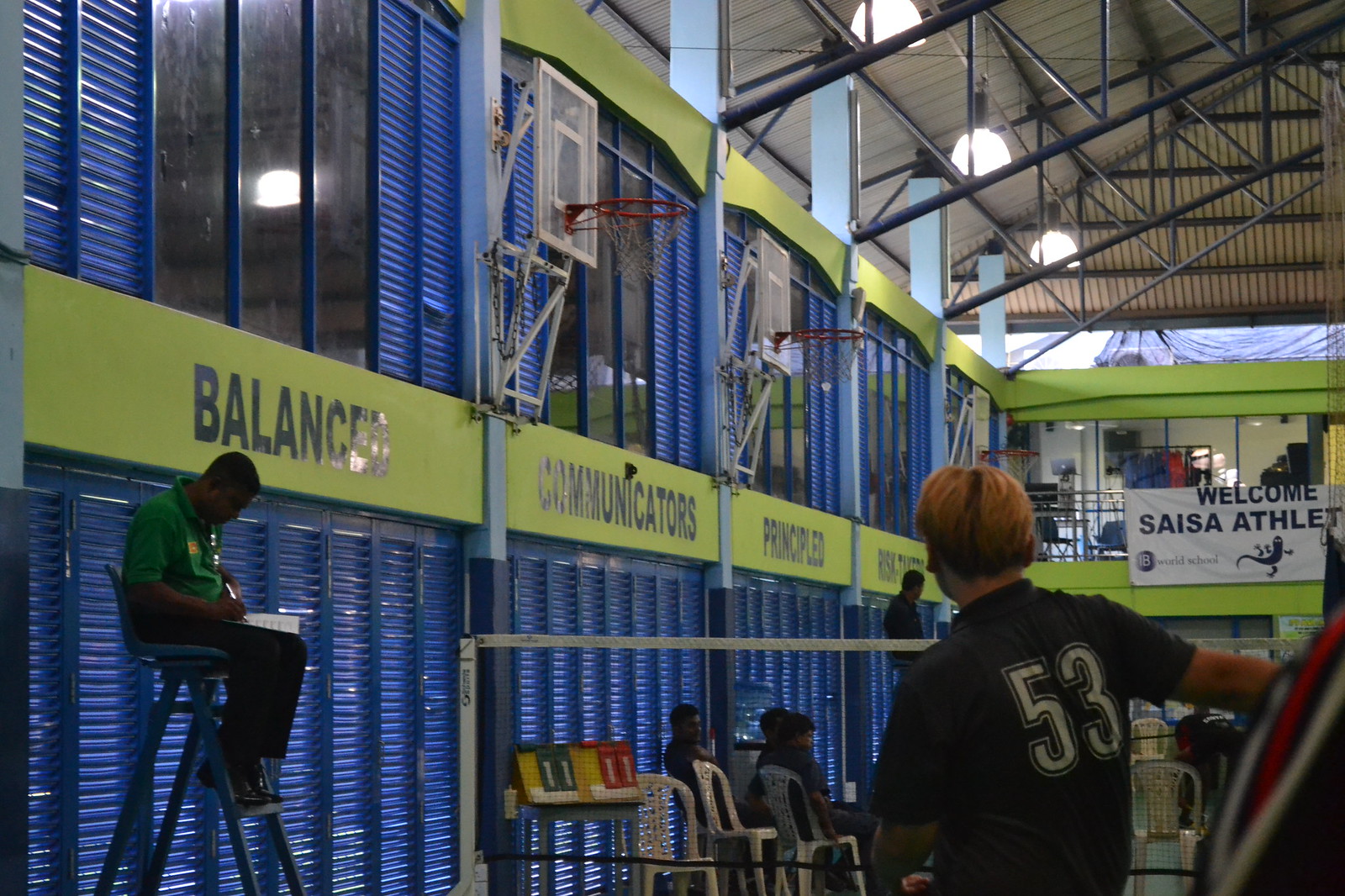The photograph captures the interior of a gymnasium featuring a multi-purpose sports court set up for volleyball, evident from the low net strung across the middle. The arena is constructed with corrugated steel walls painted blue, with a strip of yellow signage along the top bearing the words "Balance," "Communicators," and "Principals." Above the signage, three basketball hoops are folded up against the left-hand wall, not in use. Further up, between the basketball nets, there are several plexiglass windows.

In the foreground stands a man with reddish, carrot-orange hair, wearing a black t-shirt with the number 53 emblazoned in white on the back. To his left, three white plastic chairs are lined up neatly. Seated on an elevated, lifeguard-like chair to the left end of the net is another man, sporting a green polo shirt and black pants, jotting down notes. A score display device, featuring rows in yellow, green, and red, shows a tie score of 11 to 11. Across the upper right side of the gymnasium, a white sign reads "Welcome SEASA Athletes."